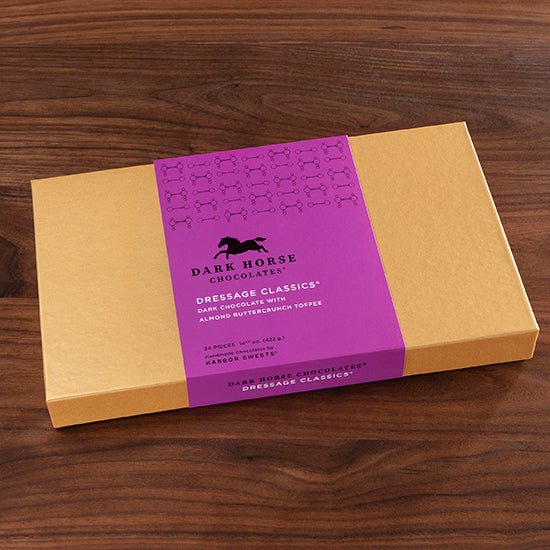The image features a light peach-orange rectangular box resting on a wooden table with visible horizontal wood grains and occasional knots. The box is adorned with a striking purple label that wraps around its front and extends to the side. At the top of the label, there are intricate black circle line designs, adding to its visual appeal. Dominating the label is a silhouette of a flying horse in black, accompanied by the text "Dark Horse Chocolates" in the same color. Below it, in elegant white lettering, it reads "Dressage Classics Dark Chocolate with Almond Butter Crunch Toffee" by Harbor Sweets. Smaller black writing provides additional details. This meticulous depiction highlights both the box's contents and its decorative elements.